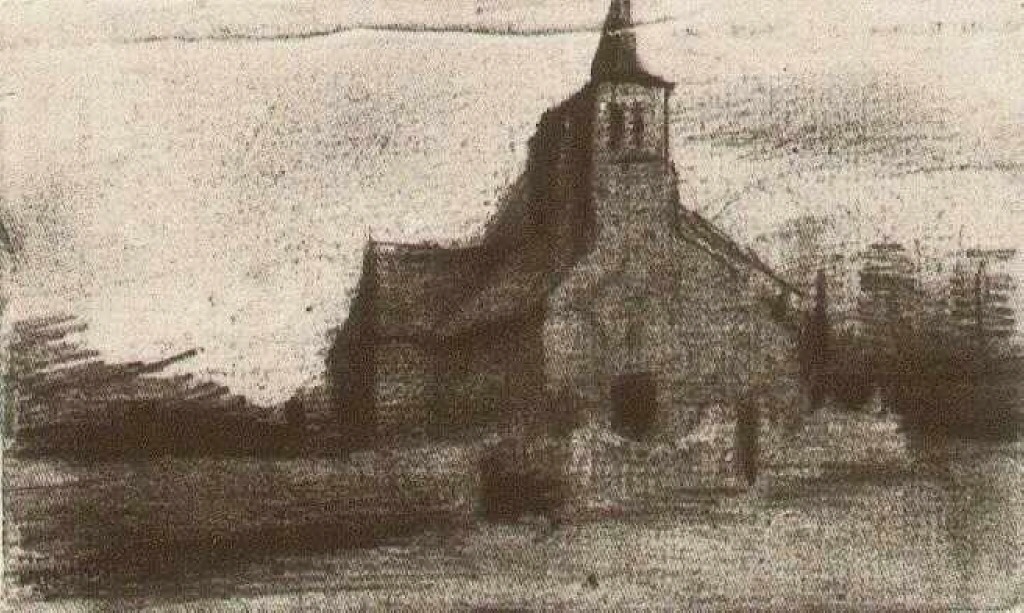This image depicts a faded, black and white sketch of an old church, primarily rendered in charcoal or a similar medium. The church, central to the composition, features a triangular roof and a prominent bell tower topped with a conical roof. Two long windows are visible on the bell tower, along with a distinct open black doorway at the front of the building. Surrounding the church are leafless trees, and directly in front of it, a low stone or cement wall with an entrance aligned with the door of the church. The area in front of the wall appears to be a flat, light-colored ground, possibly signifying a road or courtyard. The sky above is clear, without any clouds, emphasizing the stark, serene atmosphere of the scene. The sketch's quality is somewhat fuzzy, indicating age or wear, and any artist's signature present is unreadable. No people are depicted in the sketch.